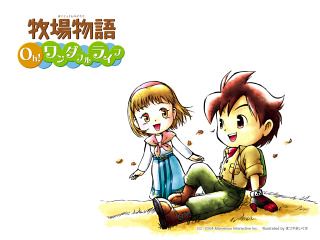The image appears to be an anime-style drawing, possibly from a cartoon or book. In the upper left corner, there are some written characters, likely in a form of Asian language, possibly Chinese, with the word "Monogatari" included. The illustration prominently features two characters, a girl and a boy, depicted in a detailed and vibrant scene. 

The girl has shoulder-length dark blonde hair with a hint of red and wears a school sailor-style uniform consisting of a blue skirt, a white blouse, and a pink necktie. Her mouth is open as if she is saying something, and she also sports a headband. She appears joyful and animated.

The boy, seated on a grassy field with his legs stretched out, exudes an adventurous spirit reminiscent of Indiana Jones. He has short brown hair and wears a beige shirt with the sleeves rolled up, green pants, brown ankle-length boots, and red gloves. He has a wide, enthusiastic smile on his face. Both characters contribute to an atmosphere of adventure and excitement, underlined by floating leaves in the background.